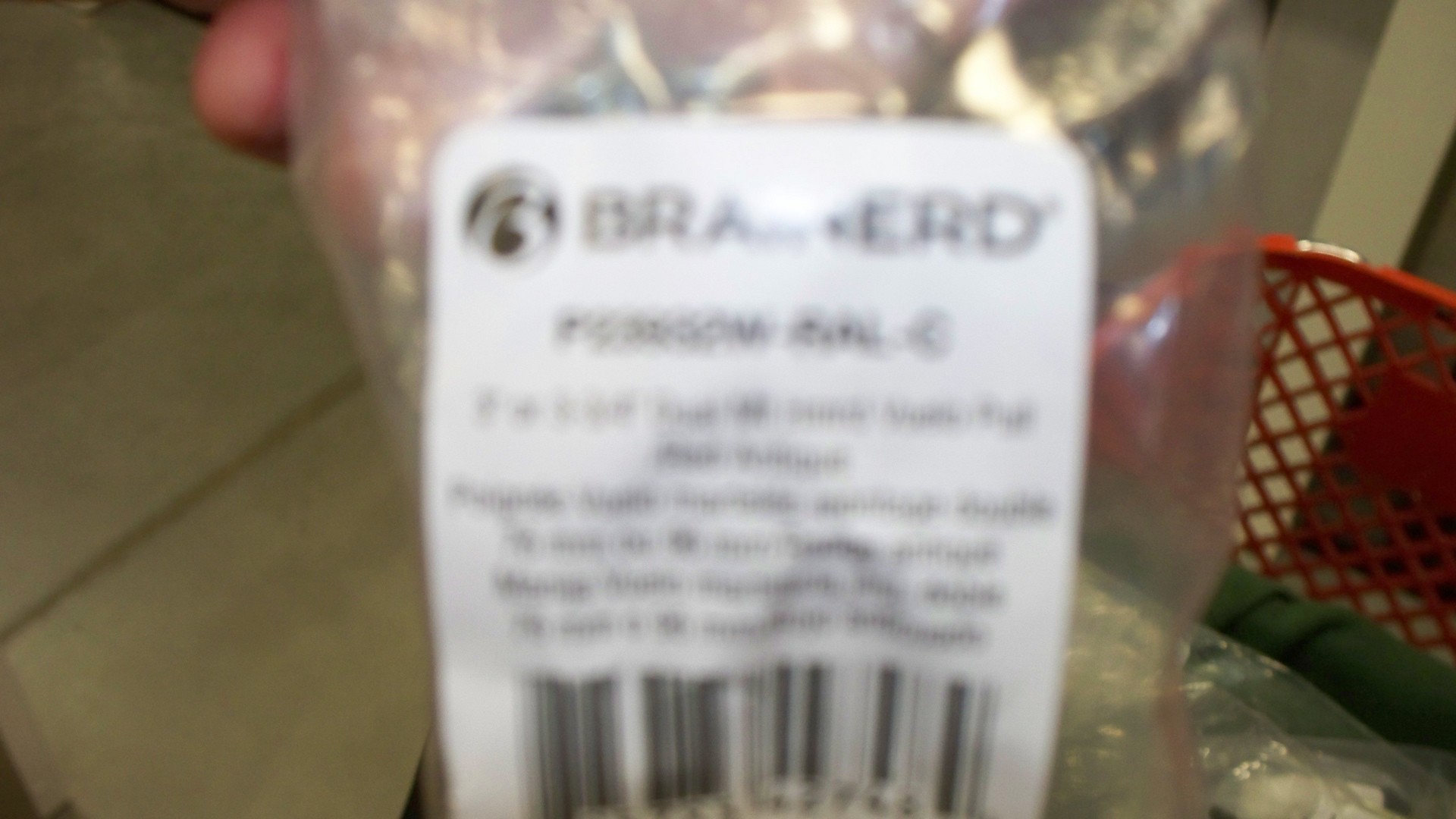The photograph captures a close-up image of a person holding a plastic-wrapped object very close to the camera, causing it to be out of focus. Through the clear plastic packaging, part of the person's fingers is visible. The plastic-wrapped item features a white label with dark brown or black font, showing partial letters that include a "B," an "R," and a "D." A black barcode is also visible at the bottom of the label, although the numbers are blurry and indistinct. In the background, a tiled floor can be seen, along with an unclear red metal object that contains a soft green item. Various surfaces in the scene reflect light, adding to the composition's overall complexity.